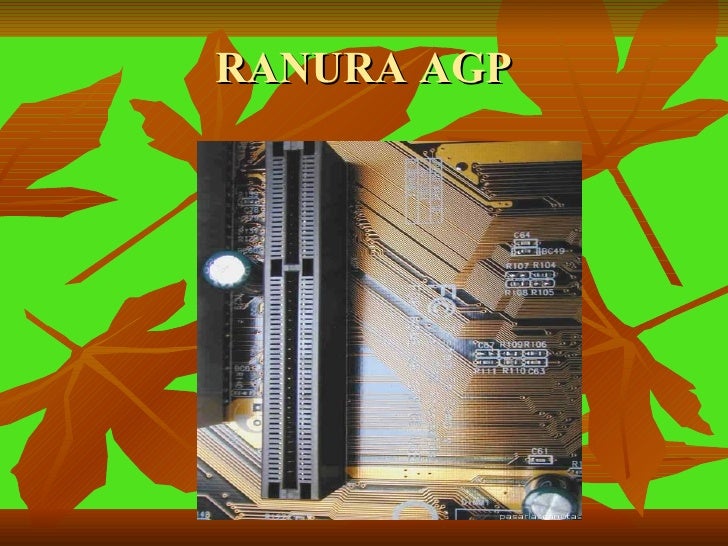The image features a detailed computer motherboard or circuitry at its center, surrounded by a textured background of brownish-red maple leaves and a green backdrop, reminiscent of a fall theme. The top of the image displays the text "Ranura AGP" in a whitish-yellow font. The motherboard itself includes tiny, unreadable writing and some discernable text like "684C64BC49" along with several semiconductors and gold circuitry. To the left of the motherboard, there's a noticeable slot likely intended for a graphics card. The image composition resembles a slide from a PowerPoint presentation, highlighted by borders: a brownish top border and a reddish bottom border. The overall color palette ranges from lime green and various shades of brown to tan, black, white, and gray, adding to the intricate and somewhat layered look of the presentation.